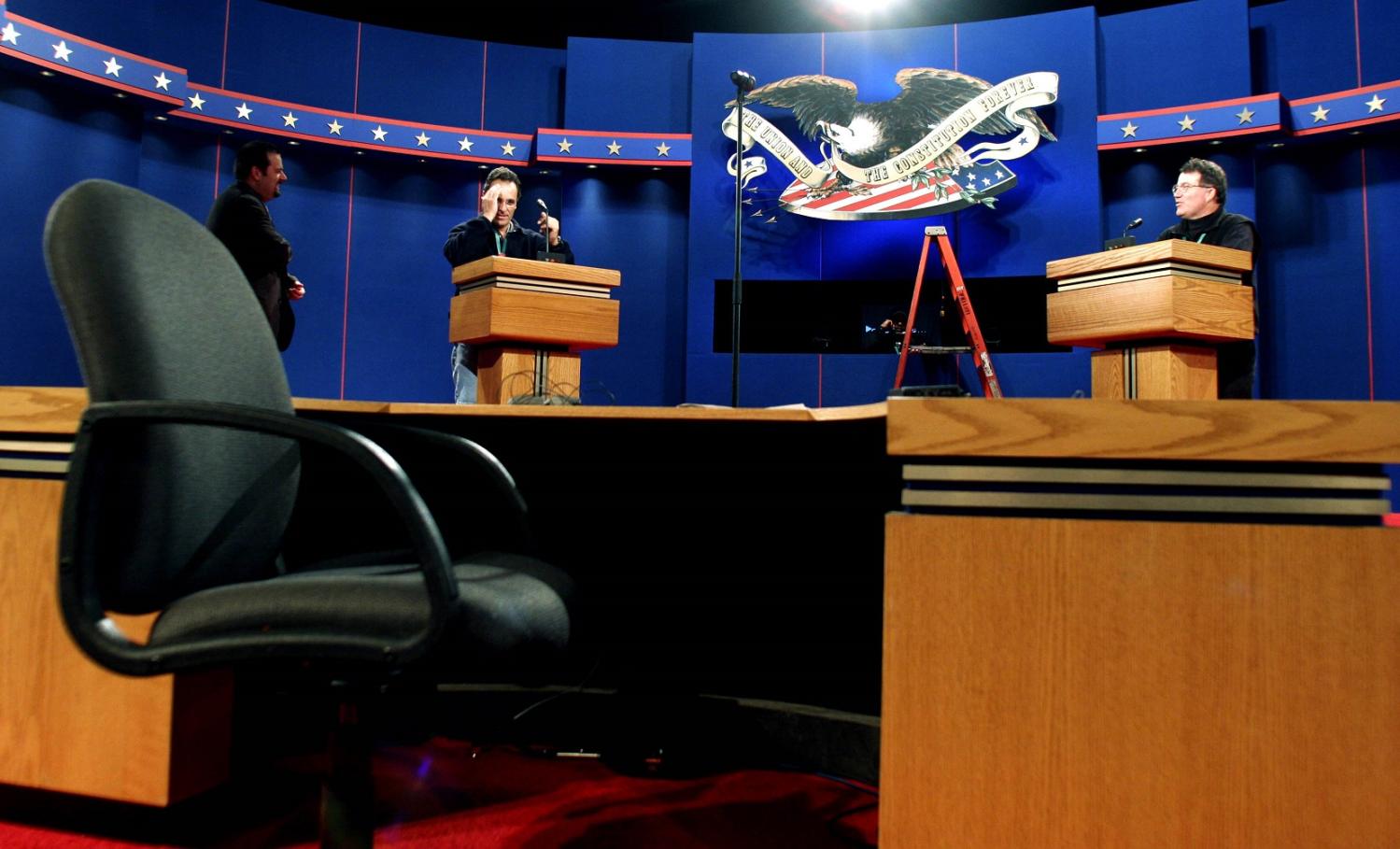The image depicts a debate stage inside a government building, possibly prepared for a presidential or leadership debate. In the foreground, there is an empty black office chair positioned in front of a brown table; this chair is likely intended for the moderator. The central focus of the stage includes two brown podiums, each with a microphone, where two gentlemen stand, apparently testing equipment. The background features a royal blue backdrop adorned with a red, white, and blue thin banner and multiple stars, emblematic of national colors. A prominent bald eagle, accompanied by the words "The Union and the Constitution Forever," is displayed centrally, emphasizing the legislative or political nature of the setting. Additionally, ladders can be seen on stage, indicating ongoing preparations for the event.